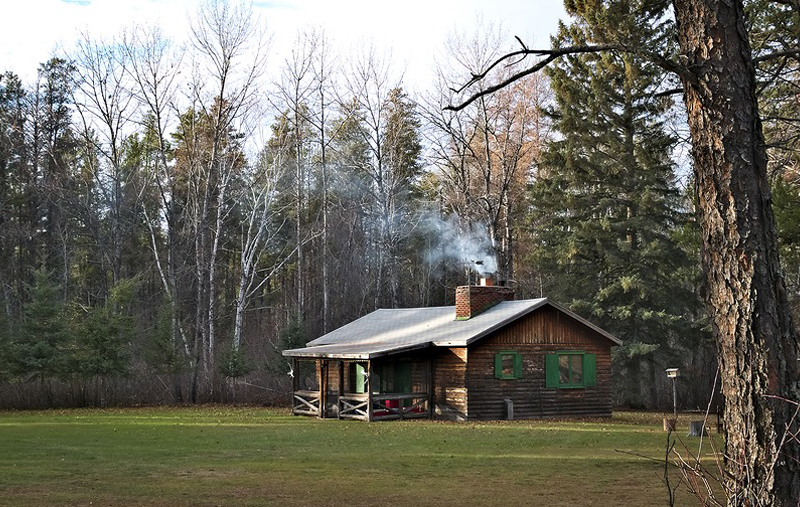This daytime photograph captures a small, aged log cabin nestled in a vast, open forest with towering trees. The cabin, constructed from dark, weathered wood, features prominent green-framed windows and a green door, which pops against the rustic backdrop. The roof of the cabin is triangular and light-colored, possibly white or light gray, and includes a covered porch at the front. On the right side of the cabin, a tall brick chimney emits smoke, suggesting someone is inside. The surrounding trees include a mix of leafy cedars and some white-barked trees that have shed their leaves. The cabin sits on a flat, grassy lawn, encircled by a fence, with a tree visible extending from the foreground. The background reveals more towering pines, and the sky overhead is cloudy yet clear, enhancing the serene forest setting.